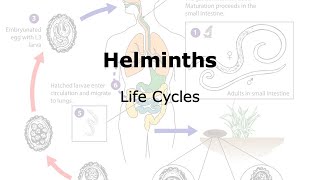The image is a small, horizontally aligned rectangle featuring the bold, black text “Helminths” at the center, with the words “Life Cycles” directly beneath in regular black font. The background contains a detailed, though somewhat faded, diagram. Starting in the lower right, circles connected by red and blue arrows curve to the upper left. In the upper left corner, next to one of these circles, there's text and a blue arrow pointing towards the top center. Here, the transparent outline of a human body is shown from the chin to the thighs, with the lungs, stomach, and intestines depicted in transparent colors: orange, green, and yellow, respectively. An additional square on the right side of the image is marked with the number one, while the number three is found in the upper left corner, indicating different stages or sections in the life cycle chart.